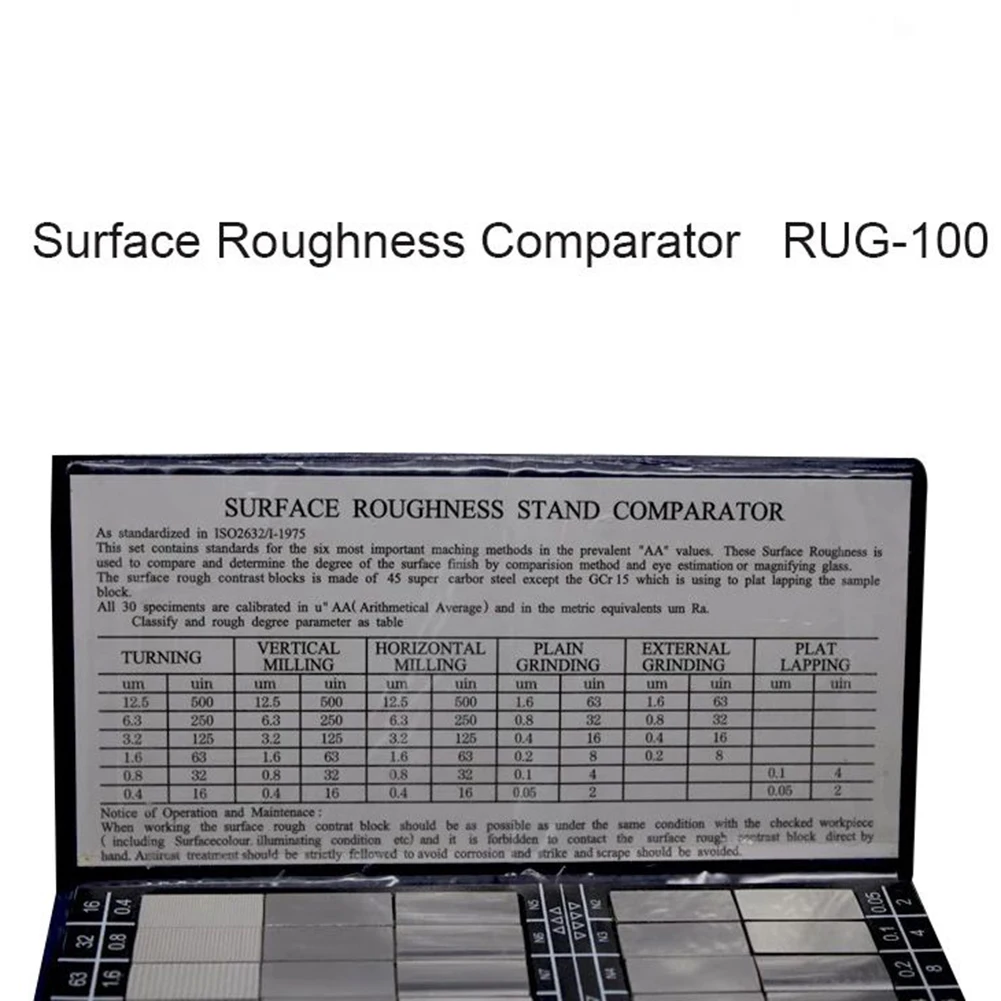The image displays a black-and-white chart titled "Surface Roughness Comparator RUG-100" on a white background with black letters. It contains a paragraph stating "Surface Roughness Stand Comparator," standardized according to ISO 2632-1-1975, detailing the six most significant methods and prevalent AA values. The chart is bordered in black, with a silver middle section, outlining 30 calibrated specimens in both UAA and metric equivalents. The chart categories include turning, vertical milling, horizontal milling, plane grinding, external grinding, and plat lapping, with corresponding numerical values. Below, the chart features various shades of silver boxes with numbers on each side, likely intended for eye estimation or magnifying glass comparison of surface roughness. The information also mentions instructions for operation and maintenance, emphasizing the tool's use in assessing and determining surface finish degrees.